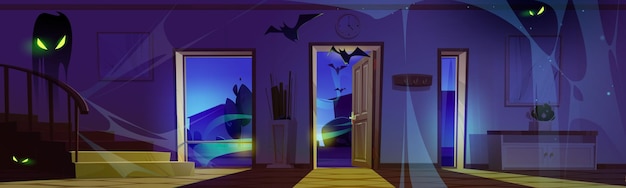This is a digitally illustrated, colored cartoon depiction of the interior of a haunted house. The scene features three open doorways in a row, with the middle door shown and leading outside where night-time darkness prevails. Two black bats are flying into the room from outside, and there are two more bats flying towards the door outside. Above the middle door, a clock reads approximately 20 minutes past midnight. Ensconced in the corners of the room are three demon-like creatures with ominously glowing yellow eyes. The predominant hues in the image are shades of purple and blue, with wood-toned effects on the floor and the curved staircase to the left. A bureau topped with a plant and a mirror above it sits within the room. The eerie atmosphere is further heightened by cobwebs or spectral goo stretching between surfaces, adding to the spookiness of the scene.